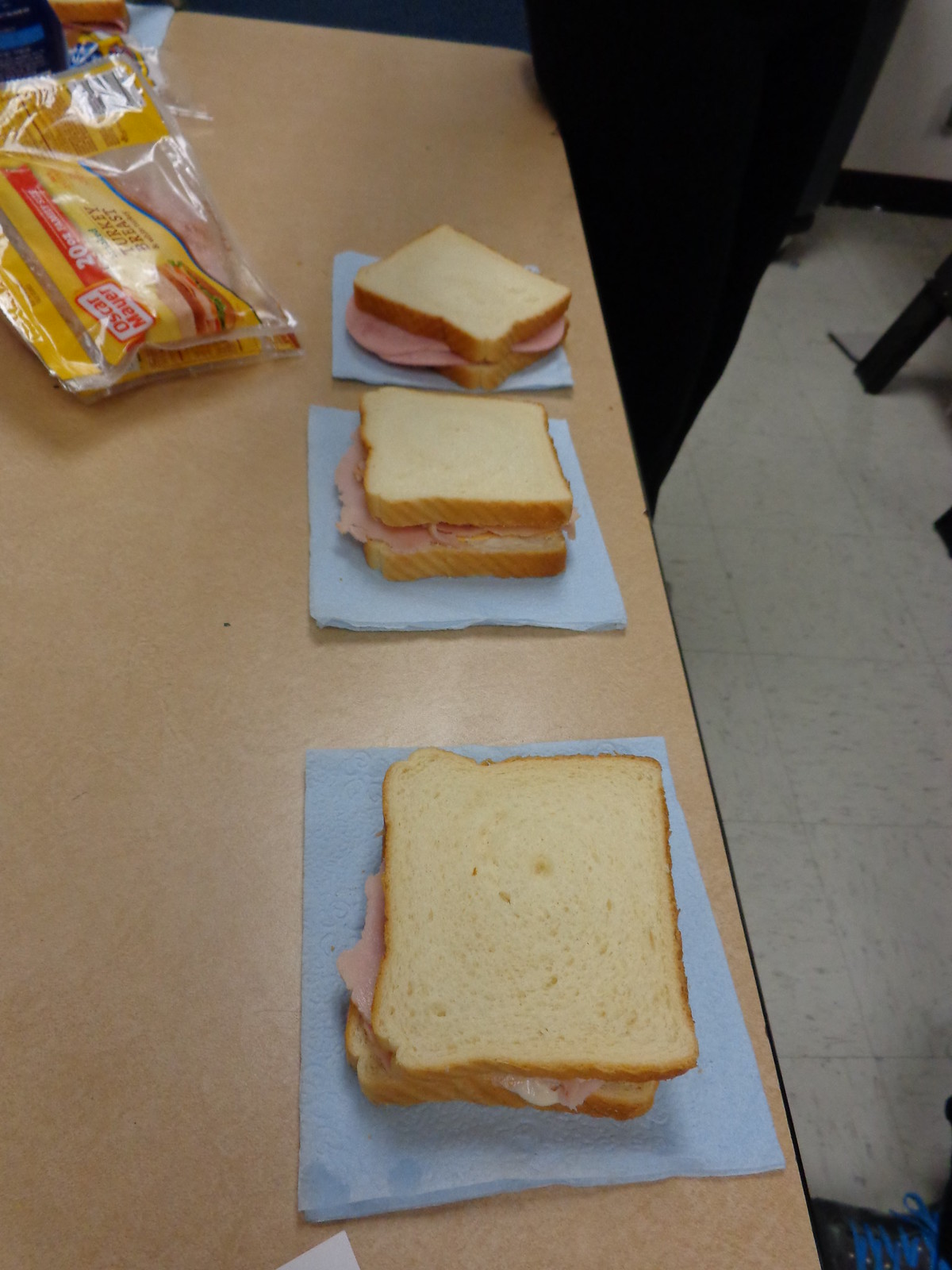The image depicts three turkey sandwiches on a long brown table with metal legs that fold in, typical of those found in schools or offices. Positioned on the right side of the table, the sandwiches are arranged vertically from the bottom of the image, with one at the top slightly angled. Each sandwich is placed on a square napkin, most likely white, though some describe them as blue. The sandwiches are made with two pieces of white bread, potentially with a slight yellowish, buttery tint. Inside each sandwich are multiple slices of Oscar Mayer turkey breast, with a large resealable bag of the turkey placed in the upper left corner of the image.

The table rests on a white tile commercial floor. In the bottom right corner, part of a person's black shoe with blue laces is visible, while another individual dressed in a black suit stands at the upper right edge of the table.